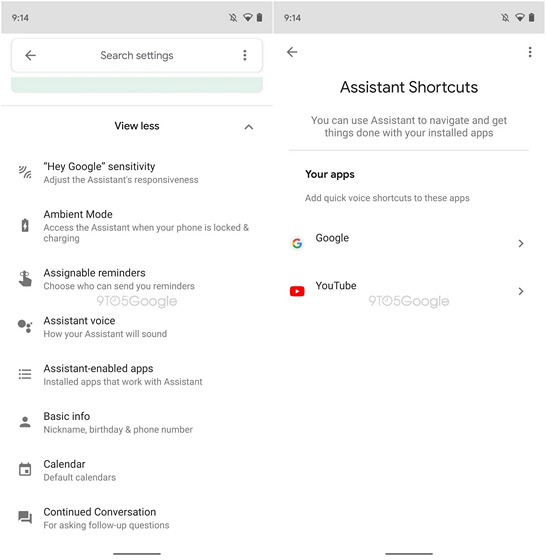The image consists of two side-by-side screenshots from a smartphone displaying Google Assistant settings. Both screenshots share identical top gray bars, showing the time as 9:14, notification silence status, consistent Wi-Fi connectivity, and identical battery levels.

The left screenshot includes a header featuring a back arrow, search settings, and a three-dot menu. Below the header, there is an option labeled "View less" with an upward arrow icon, indicating that selecting it would collapse the list of settings. The settings listed include:

- "Hey Google" sensitivity
- Ambient mode
- Assignable reminders
- Assistant voice
- Assistant enabled apps
- Basic information
- Calendar
- Continued conversation

The right screenshot displays a section titled "Assistant Shortcuts," explaining that users can navigate and manage tasks using voice commands with their installed apps. It highlights that quick voice shortcuts are configured for specific apps, listing Google and YouTube as examples. This implies that the user can initiate commands by saying "Hey Google" or "Hey YouTube" for specific actions.

The detailed breakdown contrasts the general settings overview on the left with a specific focus on actionable shortcuts on the right.